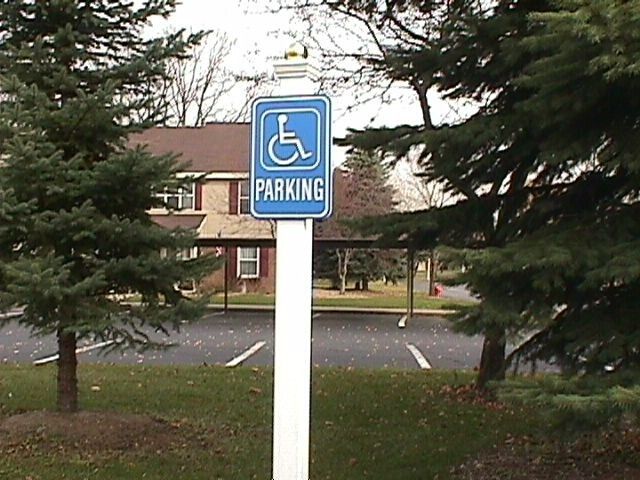In this detailed outdoor scene, a blue handicap parking sign mounted on a white pole stands prominently in the foreground. The sign features the universally recognized wheelchair symbol and is labeled "Parking" beneath the icon. This sign is set on a green median populated with a few pine and evergreen trees, some of which are either reddish or green in color. The median edges an asphalt-paved parking lot, which is empty of cars.

Behind the median, a covered walkway leads to a large, two-story brick house, featuring a front porch and framed by various trees, including a notable large tree to the right side of the house. The house is residential and appears well-maintained. The flat ground in the area is grassy with scattered fallen leaves, adding to the natural setting. In the distance to the left, a couple of other residential houses are visible. The overall scene is characterized by vibrant colors, including blue, white, green, and red, suggesting it is a sunny day, and the location exudes a serene, suburban feel.